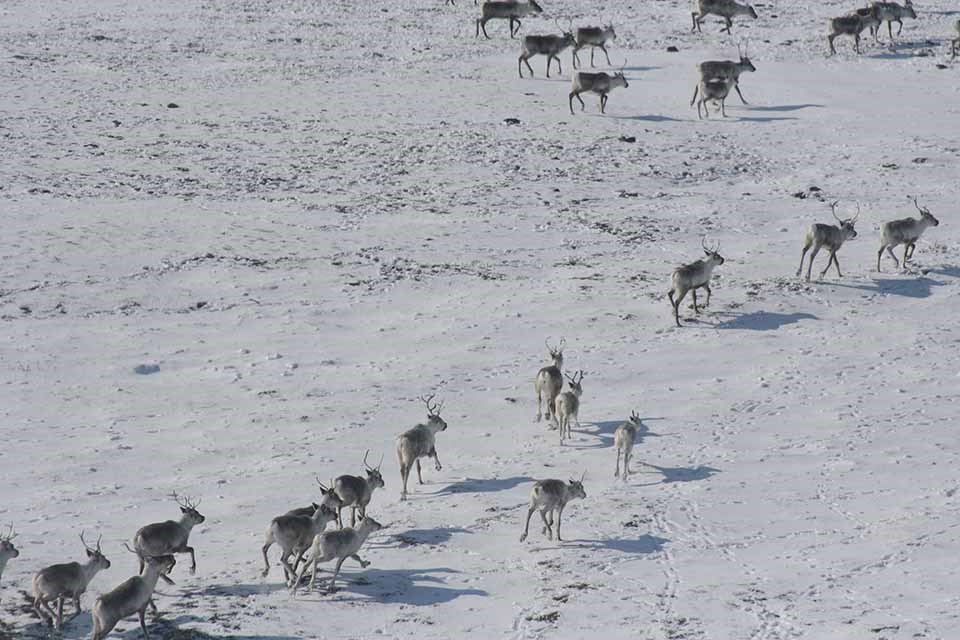This photograph captures a tranquil, snowy landscape featuring a large group of reindeer. Shot from a slightly elevated perspective, the scene showcases a thin layer of snow covering the ground, with visible footprints scattered throughout. The reindeer, numbering at least 20, create a disorganized line as they move calmly from the lower left-hand corner of the image towards the right, while a smaller cluster of them gathers at the top right-hand corner. Their prominent antlers stand out against the muted backdrop, which features patches of darker terrain contrasting with the predominantly white snow. The reindeer, appearing in shades of reddish-brown, add a sense of natural elegance to the otherwise subdued color palette of this serene winter setting.